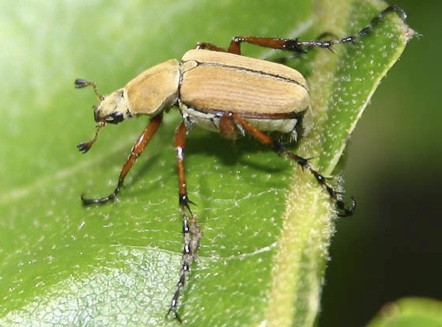This is a detailed, close-up, color photograph of a rose chaffer beetle perched on a green leaf. The image is in landscape orientation, focusing primarily on the insect, which dominates the frame. The beetle's head is facing the left side, and its tail extends toward the right side. The insect has a light brown body divided into two segments: a smaller elliptical head and a larger, more rounded lower body that exhibits a subtle black stripe running down its back.

The beetle is equipped with three long, segmented legs on each side, transitioning from brown near the body to black near the ends, with shiny dark brown portions. These legs are adorned with tiny black spikes and long hairs. Noticeably, the beetle has two dark brown antennae pointing in opposite directions. The leaf on which the beetle rests is vividly green and shiny, featuring light beige veins. The background, situated mainly to the right, is a dark green blur, making the sharply focused beetle and leaf stand out prominently.